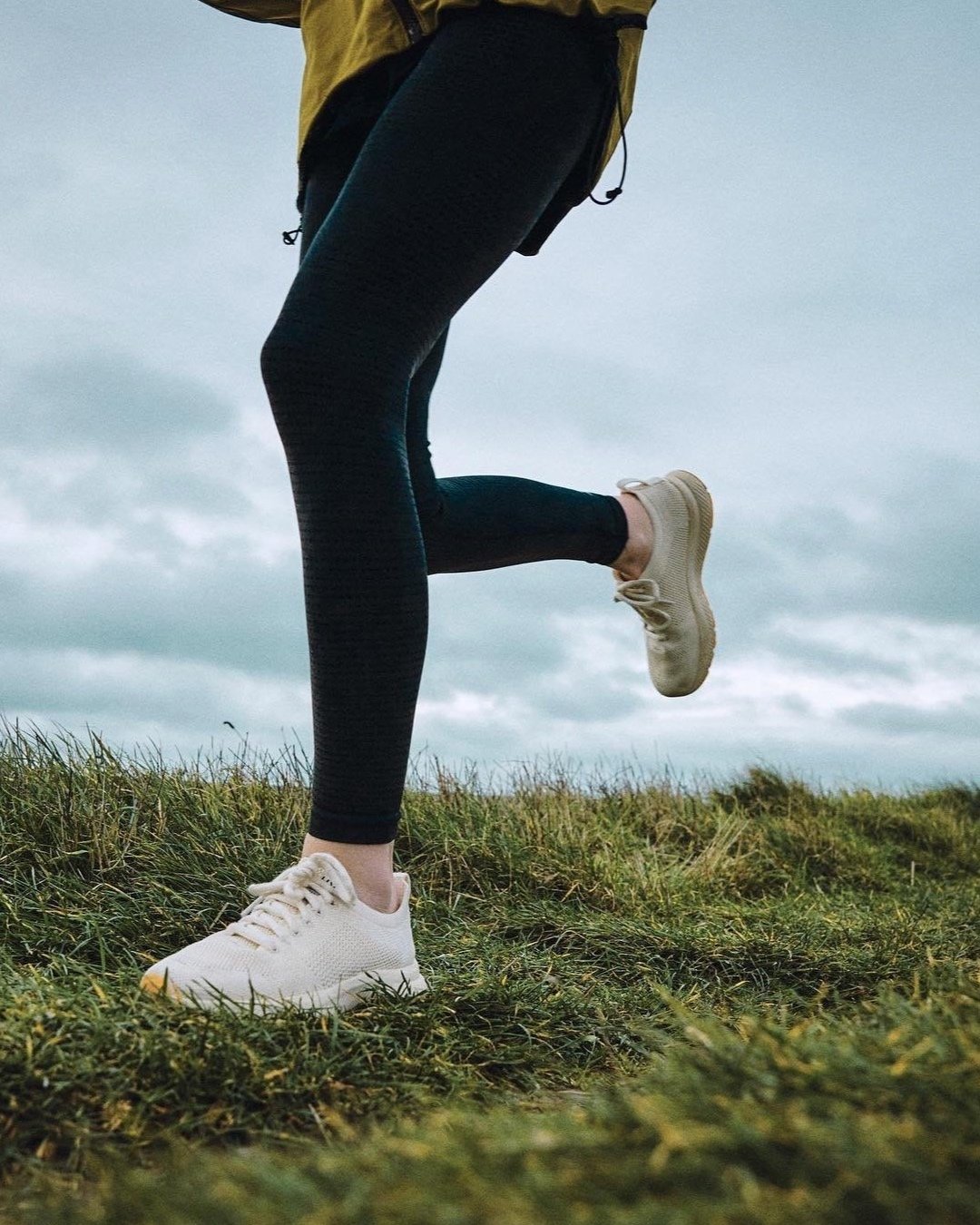This photograph captures a young lady jogging through a grassy field on a cloudy day. The scene is set outdoors, showing a stretch of dark green grass dotted with little yellow tips. The runner, dressed in a mustard-colored jacket and dark blue, almost black, leggings, moves from the right side of the frame towards the left. Her athletic outfit is completed with white tennis shoes featuring white laces, seemingly without visible socks. Her left foot is firmly planted on the trampled trail, closest to the camera, while her right leg is bent and extended behind her, indicating forward motion. Above the grass, the sky looms with gray clouds, suggesting imminent rain. The image is rectangular, roughly 5 to 6 inches high and 4 inches wide, capturing the action and the contrasting textures of the earth and sky.